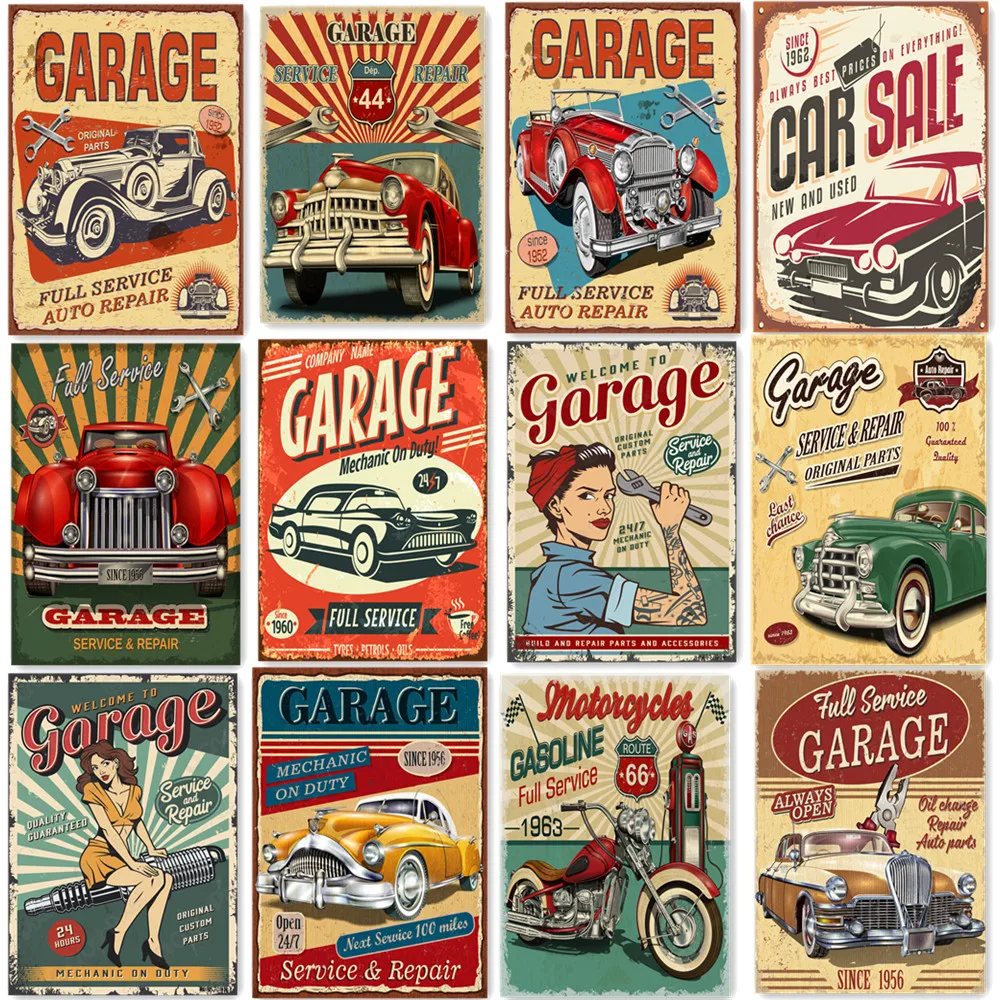The image showcases a meticulously arranged grid of 12 rectangular vintage signs, all themed around cars and garages. The layout is three rows down and four columns across, each sign adorned with vibrant colors and retro artwork. Most signs prominently feature classic cars or hot rods, with additional elements like female models, a motorcycle, and various garage-related texts.

One sign depicts a blue and white car on an orange background with "Garage" in red, reading "Full Service" underneath, and "Auto Repair" below that. Another sign, featuring red and yellow stripes at the top and a bottom blue half, displays a red car with "Garage" in black and "44" in white, flanked by "Service Repair" in blue. A similar sign pairs a red car against a yellow background, a blue square, and two crossing wrenches, alongside "Full Service" in dark brown and "Auto Repair" in orange.

The signs also include a variety of texts related to garage services such as "Full Service Garage, Always Open," "Motorcycles Gasoline, Full Service Route 66 1963," and "Service Repair Bring Original Custom Parts, 24/7 Mechanic on Duty." Notably, two signs feature female models: one stylized like Rosie the Riveter in a blue shirt with wrenches, and another woman in a red dress sitting on a giant spark plug.

Each sign boasts intricate details: one sign's background is green and yellow striped with silver crossed wrenches, another with a white and red car on a tan backdrop reads "Full Service Garage, Always Open" alongside "Oil Change, Repair, Auto Parts." The motorcycle sign has a gas pump, checkered flags, and extensive text including "Route 66" and "1963."

Overall, the artwork radiates a nostalgic charm, capturing the essence of mid-century Americana with its vibrant, vintage style.